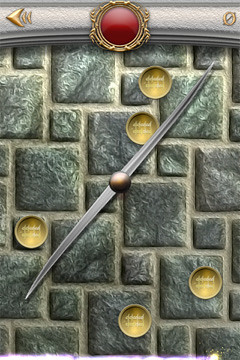The image is a vibrant, computer-generated screenshot from a video game displayed in portrait format. Dominating the center of the frame is a complex stone wall featuring a meticulous pattern of perfectly rendered square cut stones of differing sizes. Embedded within the stonework are two prominent dials that resemble an airplane propeller or clock hands. These dials, which are capable of moving in various directions, are aligned symmetrically with silver, knife-like hands extending from a brown button at their center.

Five circular gold metal discs, marked with indecipherable writing, are scattered across the stony backdrop. The background is further adorned with green tiles that add contrast to the intricate design. At the top of the image, a large red circle enclosed in a gold metallic border is observed, which likely serves as a central interactive element. To the right of this red button is a decorative golden arrow symbol, while to the left is a circle bisected by a line. Additionally, there is a back button located prominently at the top, suggesting navigation or progression functionality within the game interface. This highly detailed scene captures the immersive and intricate design typical of video game environments.